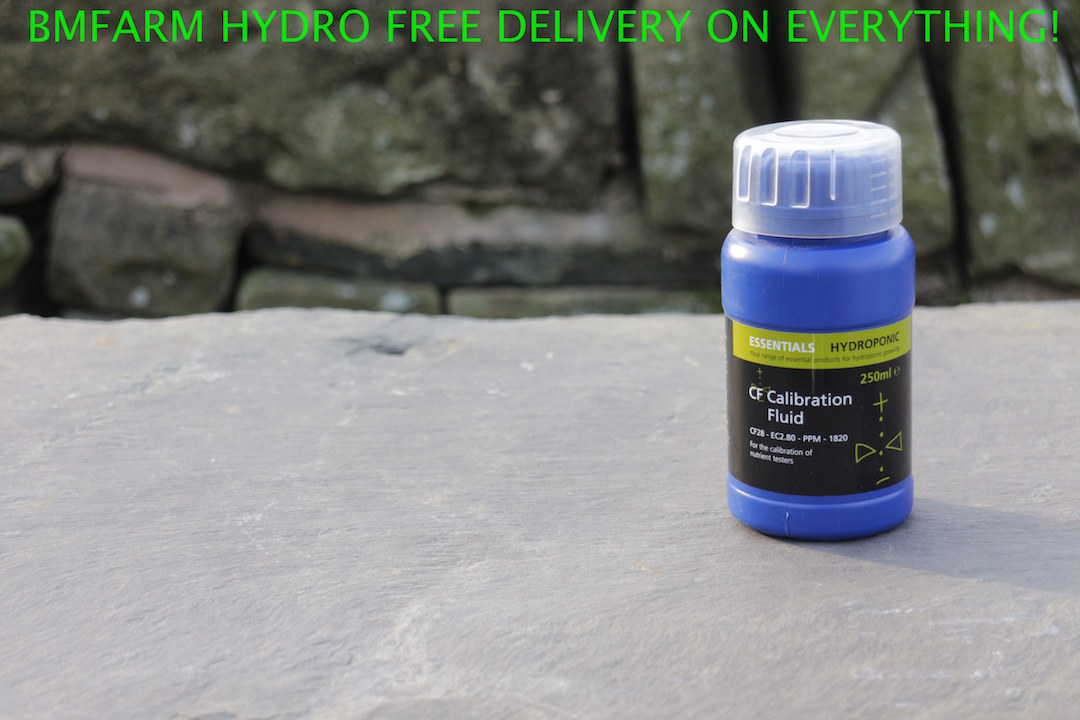This photograph features a detailed advertisement prominently displaying the text "BM Farm Hydro - Free Delivery on Everything" in vibrant lime green uppercase letters positioned at the top. The focus is on a small blue cylindrical plastic bottle with a translucent safety cap, centrally placed on a grey stone surface. The bottle exhibits a meticulously designed label: the top section, characterized by a yellow and black coloration, bears the text "Essentials Hydroponic." Below this, on a black background with white text, it reads "CF Calibration Fluid, 250 milliliters." Additional technical details, such as "CF28-EC2.80-PPM-1820," are also present, hinting at its usage in scientific or hydroponic applications. The image, taken in natural light, showcases a close-up view with a background of green stones, contributing to the earthy, outdoor setting.